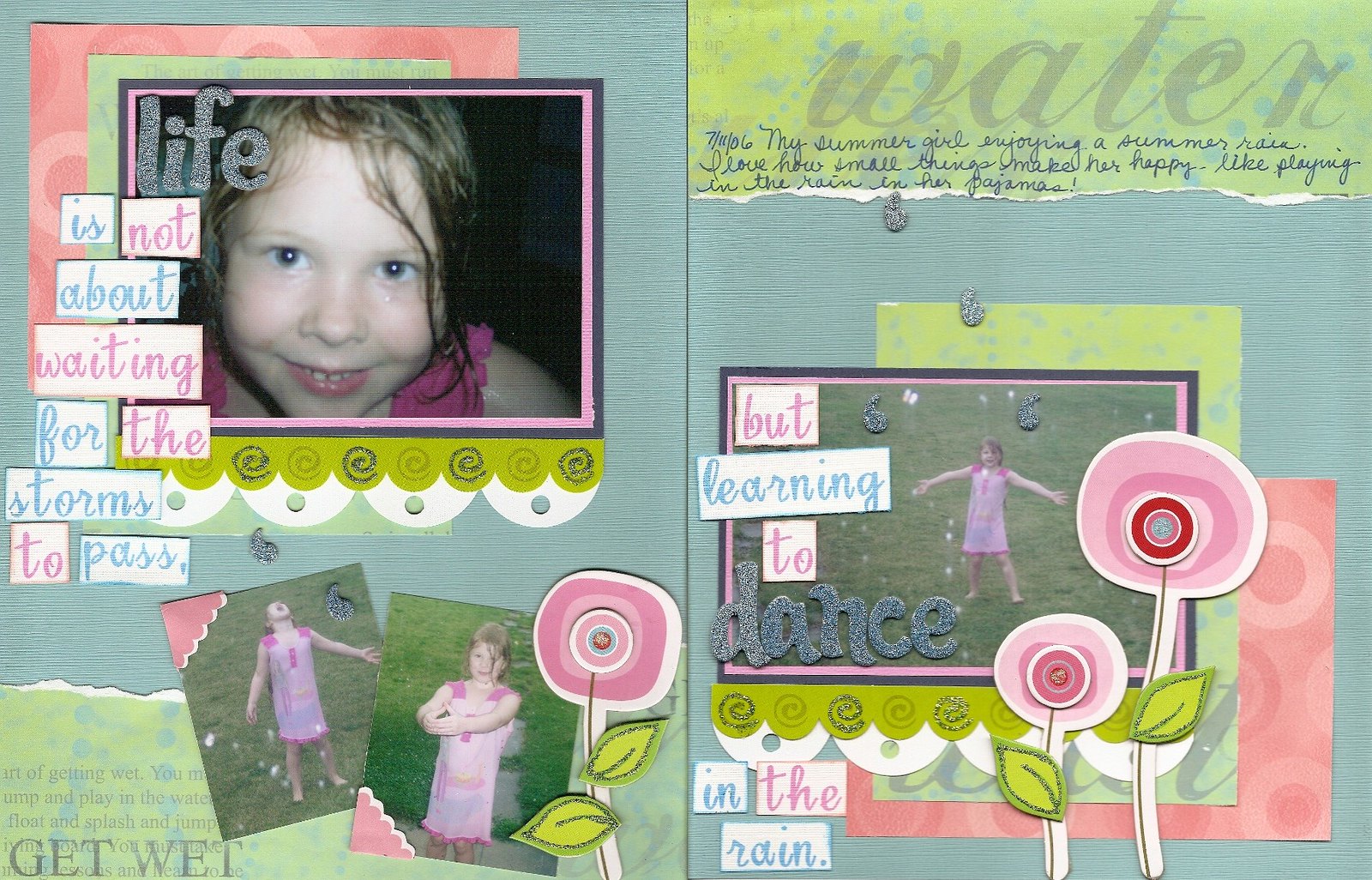This color photograph captures a beautifully designed scrapbook spread featuring a series of images and text focused on a young girl joyfully dancing in the rain. On the left page, a close-up photo of the girl's face, showcasing her long hair and pink shirt, is bordered by a pink frame. The caption around her photo reads, "Life is not about waiting for the storms to pass." Below this are two more images: in one, she stands on a lawn, looking up at the sky with her mouth open, and in the other, she reaches out her hands as if trying to cup the rain. 

The right page features another image of the girl in the same pink dress, standing outside on the lawn with her arms outstretched. The accompanying text continues with, "But learning to dance in the rain." This side of the scrapbook also includes artistic touches, such as pink flowers and pink papers thoughtfully glued over and around the photographs, reinforcing the joyful and whimsical theme of dancing through life's storms.